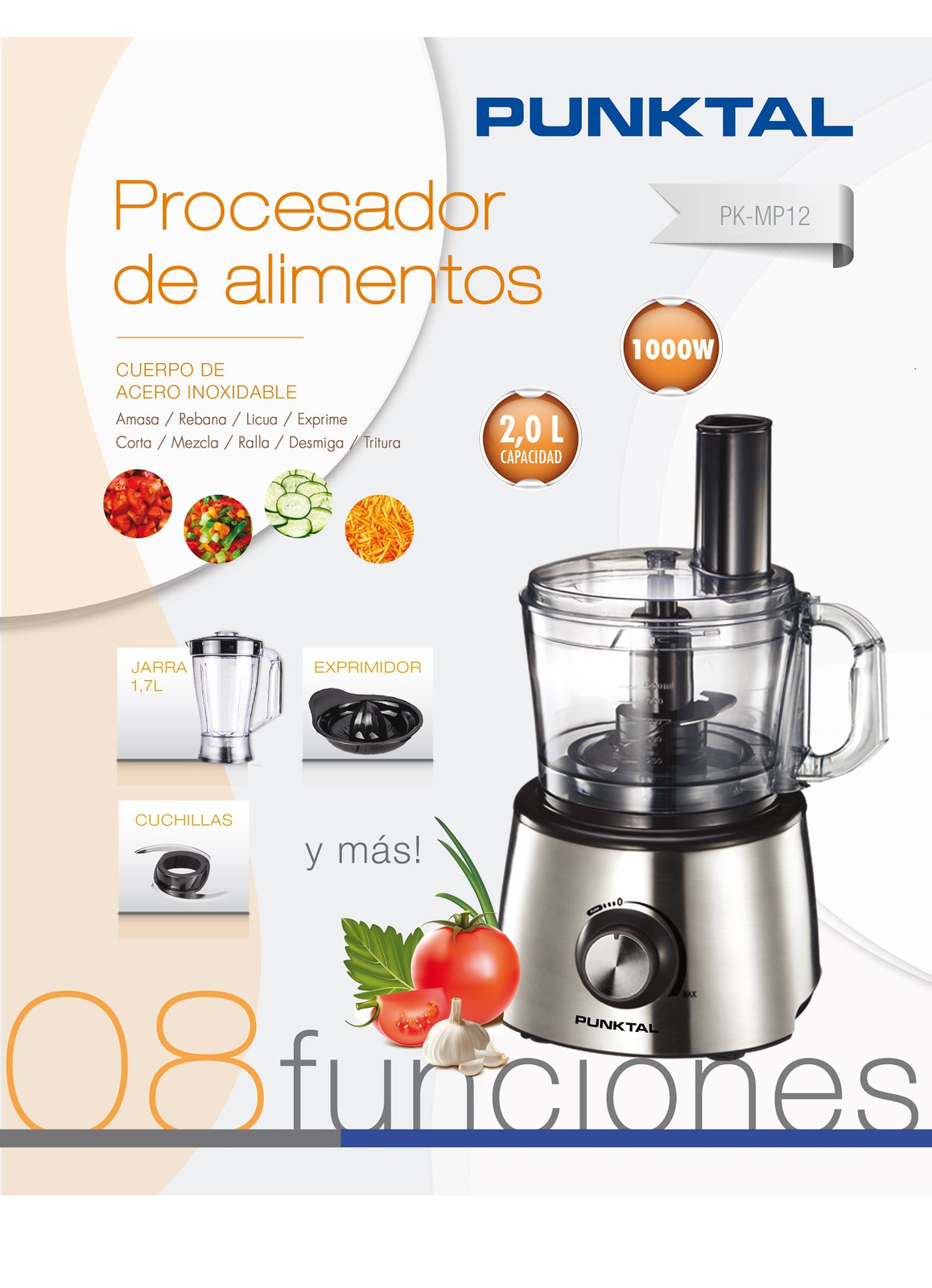The advertisement, written in Spanish, showcases a food processor from the brand "Punk Tale" in large blue lettering at the top. The white background of the ad features a curved stripe on the left-hand side. The image highlights the food processor, which has a silver base with a large dial and a clear top revealing the blade mechanics inside. A tube extends from the clear reservoir for inputting ingredients. The processor boasts 8 functions, a 2-liter capacity, and 1000 watts of power. The ad includes multiple small circular images showcasing various fruits and vegetables such as tomatoes, cucumbers, carrots, and chopped veggies, indicating what the processor can handle. Additionally, the photo displays different attachments and components, including a blender and a possible juicer. At the bottom left of the image, there are pictures of tomatoes, garlic, and a leaf, further emphasizing the processor's versatility.